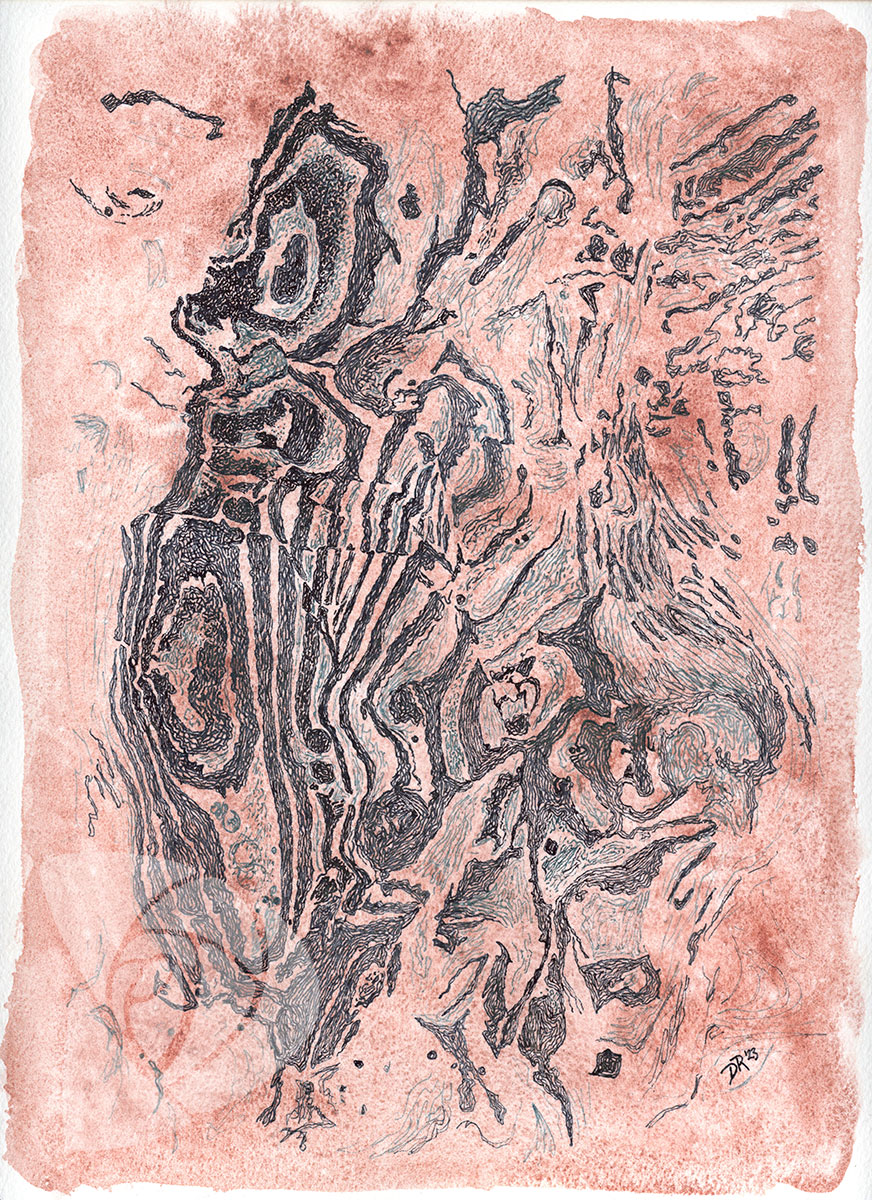This image showcases an abstract piece of watercolor art on white paper, with a predominantly pink or rose background that fades towards the edges, giving it a soft, ethereal appearance. The central focus is an intricate composition of black and gray lines and squiggles, reminiscent of a contour map and applied with what appears to be a fine ink instrument. The black ink is denser towards the right side and lightens as it spreads out, adding depth to the abstract design. There is also a small detail of a faint red watercolor on the lower left corner. The canvas is more vertical in orientation, and near the bottom, one can observe the artist's initials or name signed as "DR23."